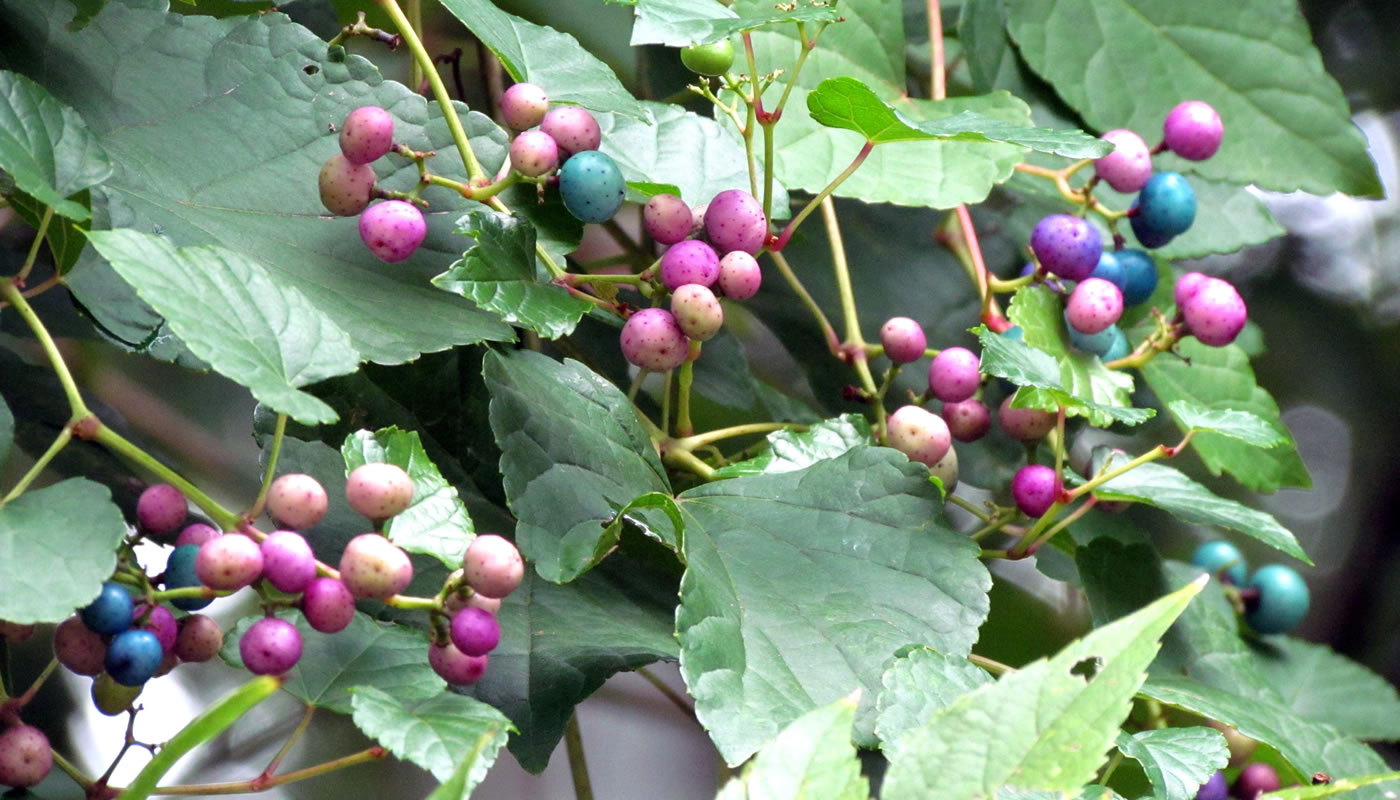The image features a close-up view of a lush bush adorned with an assortment of vibrant berries at various stages of ripeness. The foliage is a rich green, creating a lively backdrop for the berries, which exhibit a spectrum of colors ranging from beige and green to pink, purple, and blue. This colorful array suggests that the berries are in different stages of development, with some appearing almost ripe while others are just beginning to mature. The primary focus is on the berries and leaves, rendered in sharp detail, while the background is beautifully blurred with a bokeh effect, emphasizing the bush’s place in a sunlit, garden-like setting. One can notice a cluster of round berries, and a particularly noticeable green grape-like berry near the frame's border, adding to the image's intricate detail. The overall impression is that of a vibrant, sun-drenched scene, possibly a snapshot from a farmer's garden during the mid-growing season.